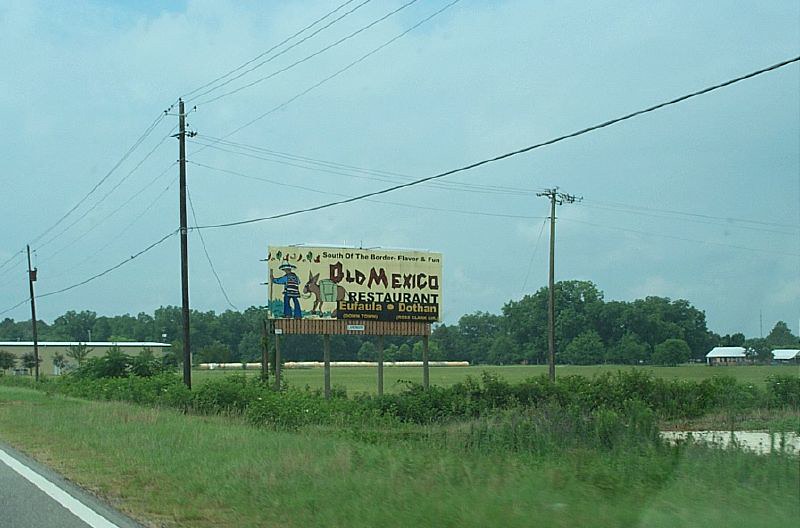This image captures a vivid roadside scene featuring a large, prominent billboard on the side of a highway. The billboard stands on four wooden posts amid lush vegetation, including dense green bushes and high-reaching leaves right underneath. The sign has a striking yellow background with an illustration of a man in a sombrero walking leftwards, leading a brown donkey behind him; the donkey is adorned with light green tack. The billboard promotes an "Old Mexico Restaurant," with a tagline reading "South of the Border Flavor and Fun," while also mentioning "Unifala Tothan." Above and beside the billboard, several power lines intersect the sky. The foreground includes a strip of road with a visible white line and patches of green grass that lead off towards the left. In the background, to the left and right of the vegetation, there are farm buildings with brown exteriors and one distinct building with a white roof. Further back, a dense line of trees stretches across, their foliage thick and vibrant, completing the picturesque rural setting.